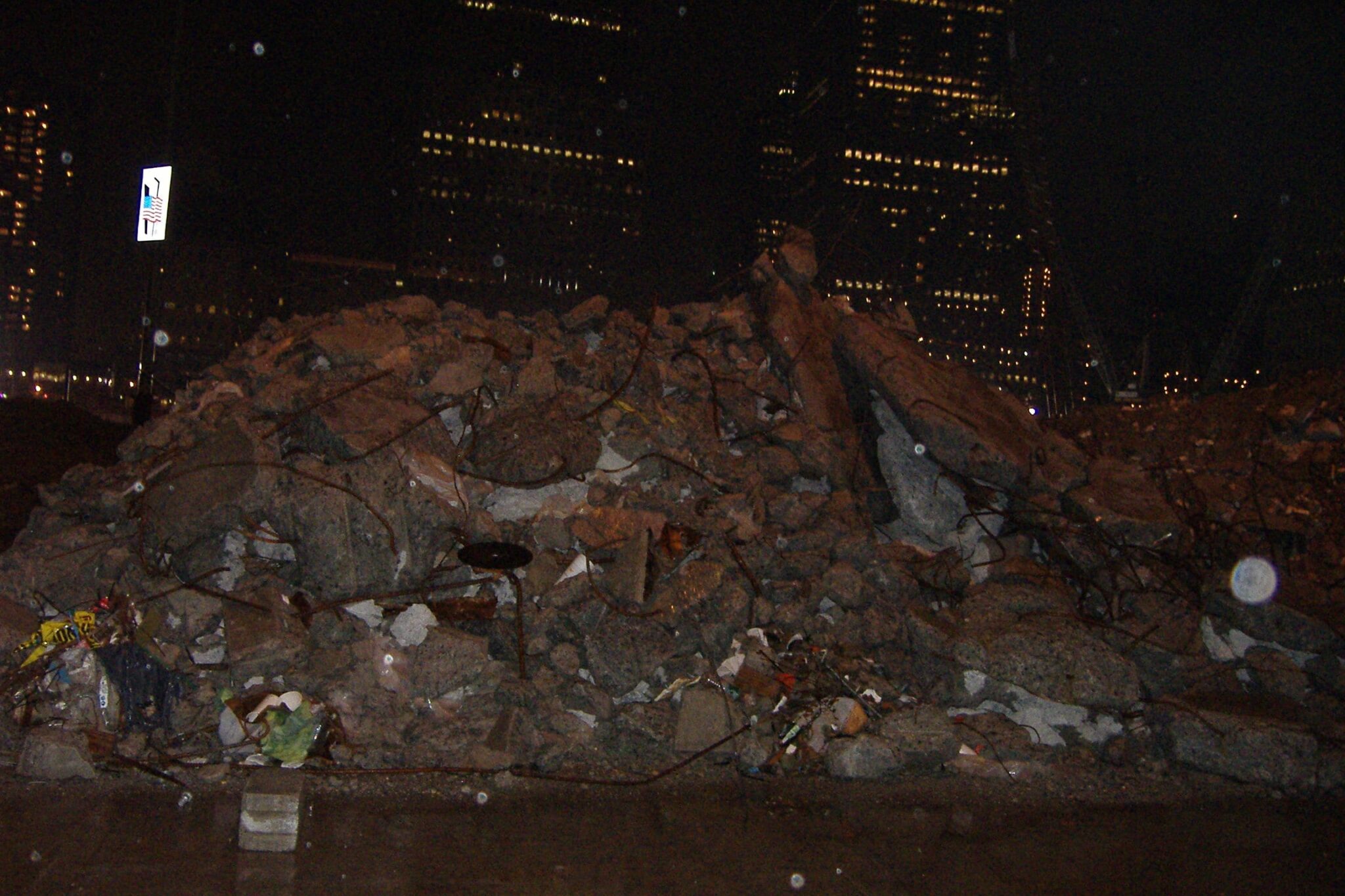This nighttime photograph captures a towering pile of rubble, possibly from a collapsed building or demolition, situated prominently in a cityscape. The heap is massive, filled with various materials including concrete chunks, twisted rusted rebar, pipes, and scattered trash. Yellow caution tape and brick fragments are also visible amidst the debris. The scene is set against a backdrop of illuminated skyscrapers, their many lit windows piercing through the darkness, highlighting the scale of the urban environment. A bright white light to the left also features an American flag, indicating the location is likely in the United States. The ground in front of the rubble has a noticeable sheen, suggesting either wet conditions or recent rain, adding a reflective quality to the nighttime setting.